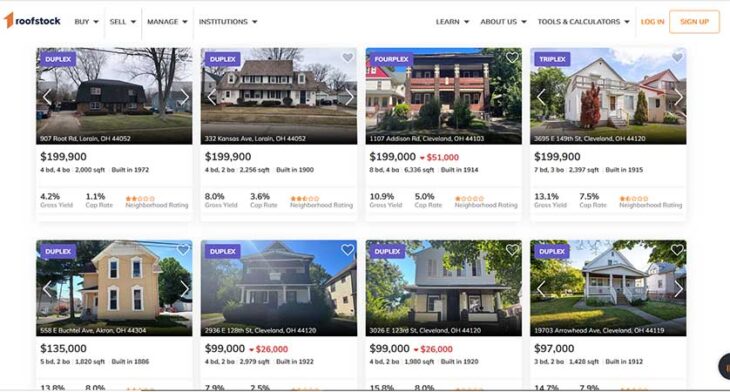Screenshot of a website displaying real estate listings on a desktop interface. At the top, the website name, "Roofstock," is prominently featured with options to "Buy," "Sell," and "Manage," targeted towards institutional investors. Each option is accompanied by a drop-down arrow for further navigation. On the right-hand side, there are links to "Learn About Us" and "Tools and Calculators," both also featuring drop-down arrows. Additionally, there are buttons to "Log In" or "Sign Up."

Below this header, two rows of home listings are visible. 

The first property is a duplex located at 907 Sutton Road, Lorain, Ohio, priced at $199,900. It features 4 bedrooms and 4 bathrooms, spanning 2,000 square feet, and was built in 1972. The listing shows a 4.2% (unreadable) and a 1.1% comp rate. The neighborhood is rated 2 out of 5 stars.

The second property is another duplex situated at 322 Kansas Avenue, Lorain, Ohio, 44052. It is also priced at $199,900, with 4 bedrooms and 2 bathrooms, covering 2,256 square feet, constructed in 1998. The property boasts an 8% gross yield and a 3.6% comp rate. The neighborhood has a rating of 2.5 out of 5 stars.

The third listing is a four-plex located at 1107 Addison Avenue, Cleveland, Ohio, 44103. Further details are not visible in the screenshot.